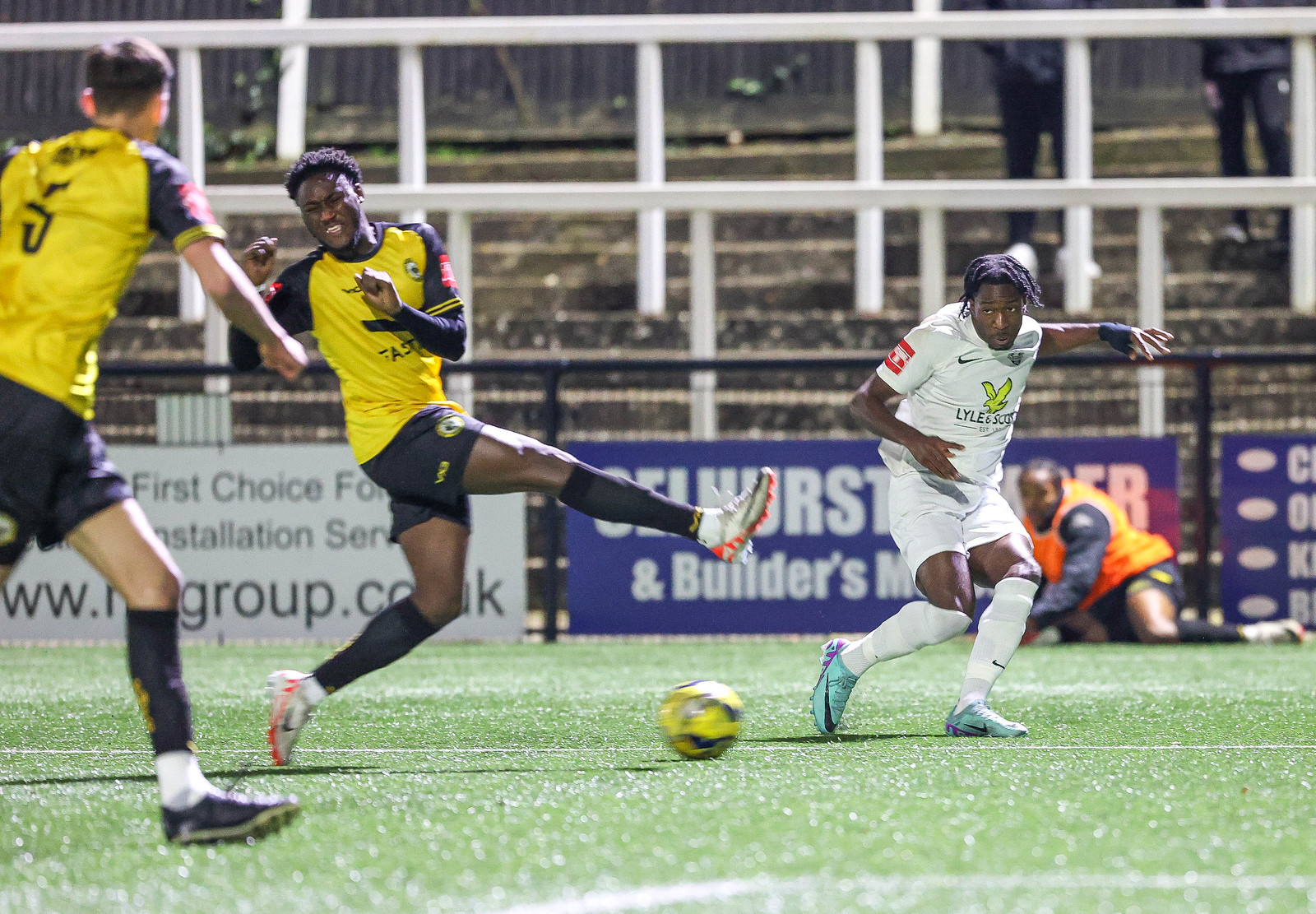In this dynamic and action-packed soccer match photograph, we see a crucial moment captured in mid-action. On the right side of the image, an opponent dressed in an all-white uniform, with a logo that reads "Lyle" and an insignia of a yellow bird on their chest, is running forward. Their gaze is intensely focused straight ahead. The soccer ball, yellow and slightly blurry in motion, is coming towards this player, indicating it has just been kicked. Behind the ball, a player dressed in a black and yellow jersey, with black shorts, white shoes, and black socks, is caught in the act of kicking, their right leg extended mid-air, demonstrating a powerful kicking motion with their body twisted. This player is African-American, with a look of concentration on their face. In the foreground, partially blurred, another teammate wearing the same black and yellow uniform is visible, distinguished by the number 5 on their back. This teammate is facing away from the viewer, contributing to the sense of movement and intensity in the scene. The contrasting attire and the players' dynamic poses emphasize the competitive nature of the game.